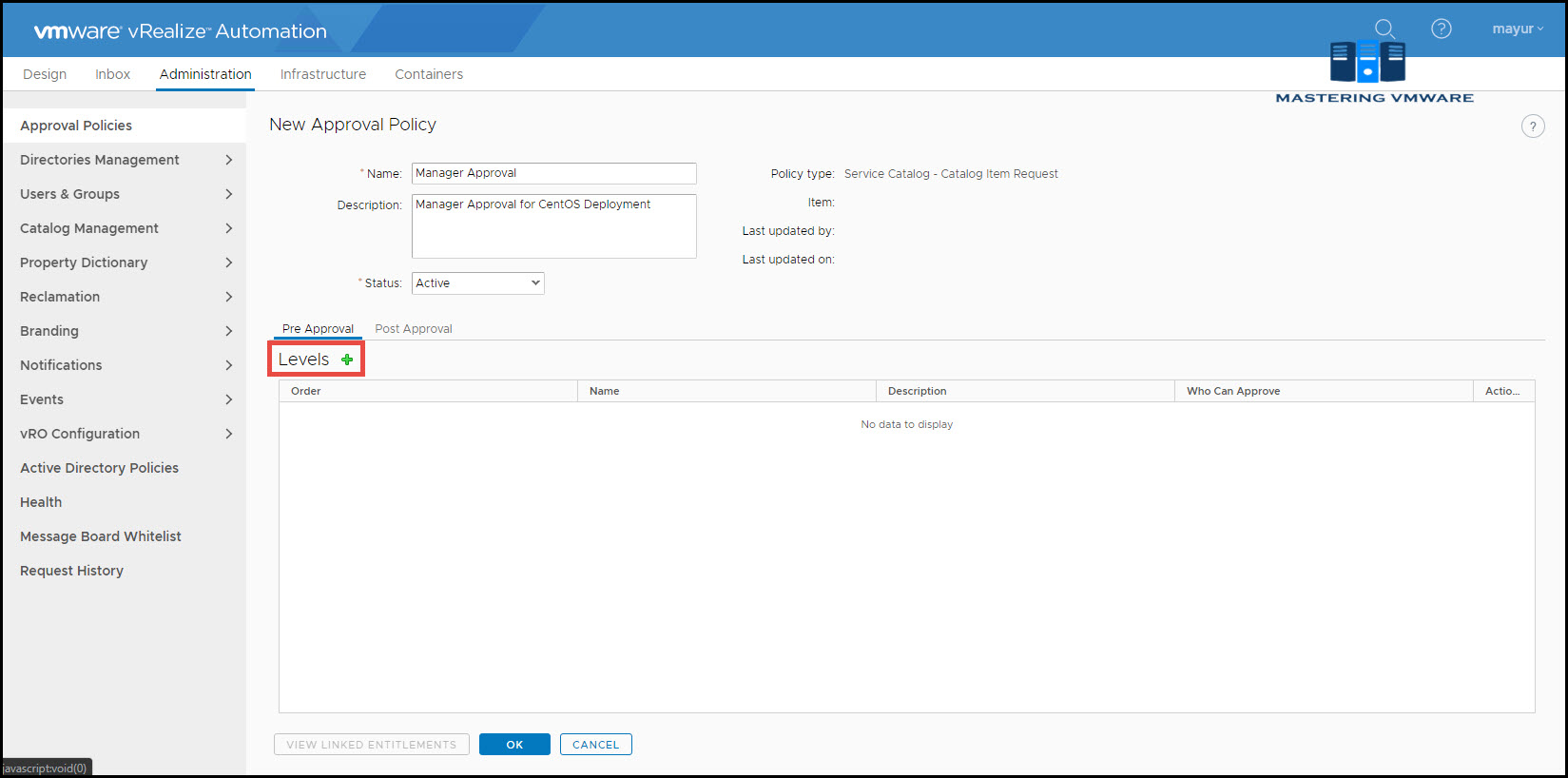A screenshot of a VMware vRealize Automation web page, characterized by a blue header featuring the software's name with a faint capital "V" in the background. Below the header, navigation links for "Design," "Inbox," "Administration," "Infrastructure," and "Containers" are visible. On the left side, a menu lists various sections including "Approval Policies" (the current selection), "Directories," "Management," "Users and Groups," "Catalog Management," "Property Dictionary," "Reclamation," "Branding," "Notifications," "Events," "VRO Configuration," "Active Directory Policies," "Health," "Message Board Whitelist," and "Request History." The central area contains multiple interactive fields, with a red box highlighting the word "Levels."